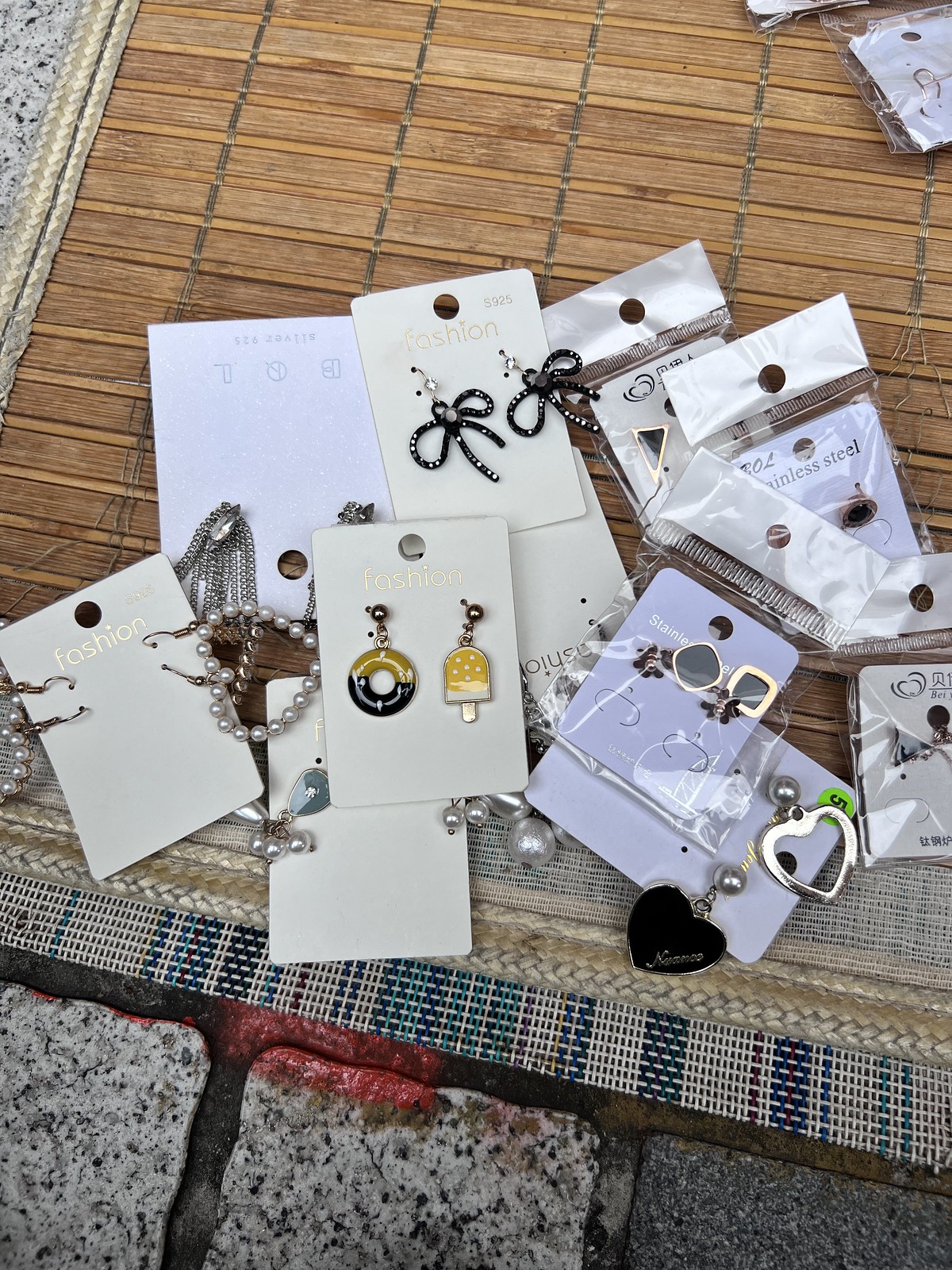This image depicts a bamboo rug with a tweed trim laid out on square stone blocks with thick lines of grout in between. On the rug, there is a diverse collection of earrings, many still attached to their plastic backing or enclosed in plastic wrapping. The earrings range in design, including hearts, black bows, and playful motifs such as a gold popsicle, a black and gold donut, and an ice cream paired with a donut. Some of the earrings are made of pearl-like material and subtly blend into the arrangement of jewelry, which is densely scattered, with some pieces stacked on top of each other. A few earrings situated in the upper right corner are partially cut off, making their details indiscernible. Towards the edge of the rug, there is a red substance that appears to have spilled at some point. Overall, the jewelry consists of smaller, more delicate pieces, with several marked as stainless steel, showcasing a variety of intricate styles.